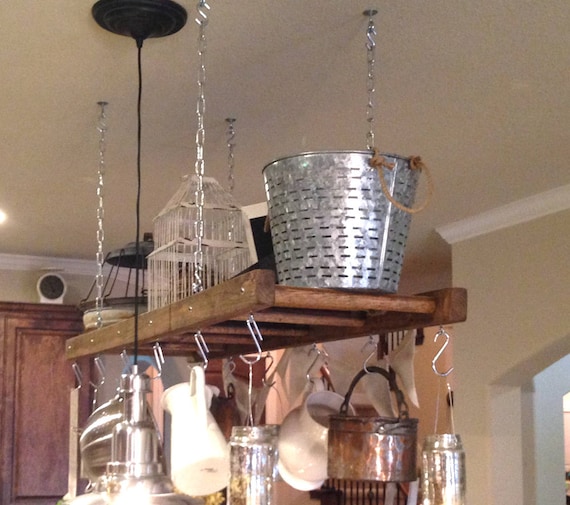The image depicts a wooden ladder, repurposed as a decorative kitchen pot rack, suspended by four silver chain links in the middle of a kitchen. The ladder, hung horizontally, is accompanied by various items: a stainless steel bucket with a rope handle at the end, a white birdcage positioned centrally, and a slotted stainless steel bucket, which suggests a utility for straining or rinsing food items. The ladder itself features multiple S-hooks from which an assortment of kitchen utensils, metal buckets, carafes, and mid-century style kitchenware are suspended. The background reveals an off-white painted ceiling and walls, a woodgrain cabinet with either a camera or light fixture placed on top, and an arched doorway to the right. Additional kitchen accessories, some reminiscent of mid-century design, augment the eclectic yet functional aesthetic of the space.